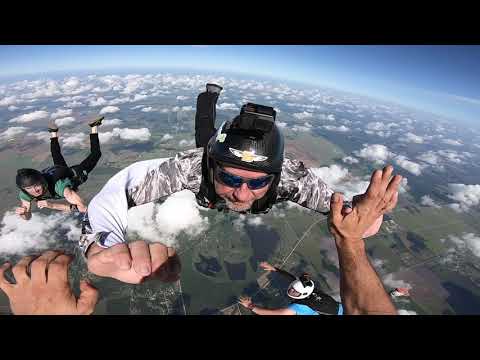A thrilling aerial scene captures four skydivers in mid-air, set against the backdrop of a clear blue sky and white fluffy clouds. The perspective is from one skydiver whose outstretched hands face another man directly in front of him. This central figure, an older man with a white beard, is sharply painted in a white long-sleeved shirt adorned with gray designs, a black helmet mounted with a black camera, and eye protection. His right hand grips the outstretched hand of the camera holder, while his other hand remains free. To his left is another skydiver dressed in a green shirt and black pants, also wearing a black helmet. The scene captures the immense altitude with the ground far below, a green canvas with patches of blue water, adding a sense of grandeur and scale to this exhilarating moment.